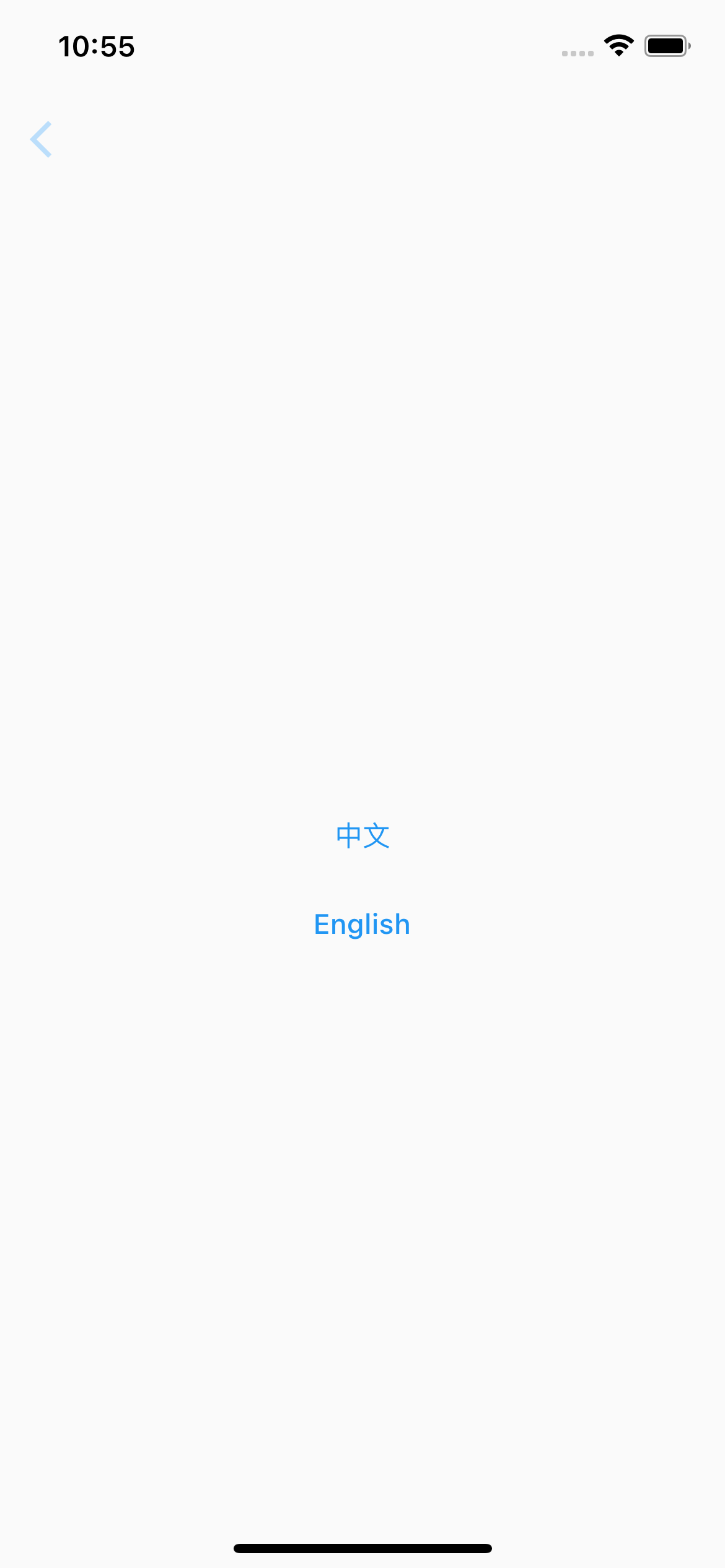This is a vertically rectangular screenshot from a cell phone. The background is a light gray color. In the upper left-hand corner, the time "10:55" is displayed in bold black font. In the upper right-hand corner, a filled-in black battery icon is visible, situated next to triangular Wi-Fi signal bars.

About two lines below the time on the left edge, there is a light blue arrow pointing to the left, resembling a sideways "V." Slightly below the center of the screenshot, two light blue Chinese symbols are displayed, centered horizontally. The symbol on the left is a rectangle with a vertical line through it, while the one on the right looks like an upside-down triangle with an upside-down "V" extending from its bottom.

Approximately three lines below the Chinese symbols, the word "English" is centered and displayed in the same light blue color. At the very bottom of the screen, a thick, bold black horizontal line is centered.